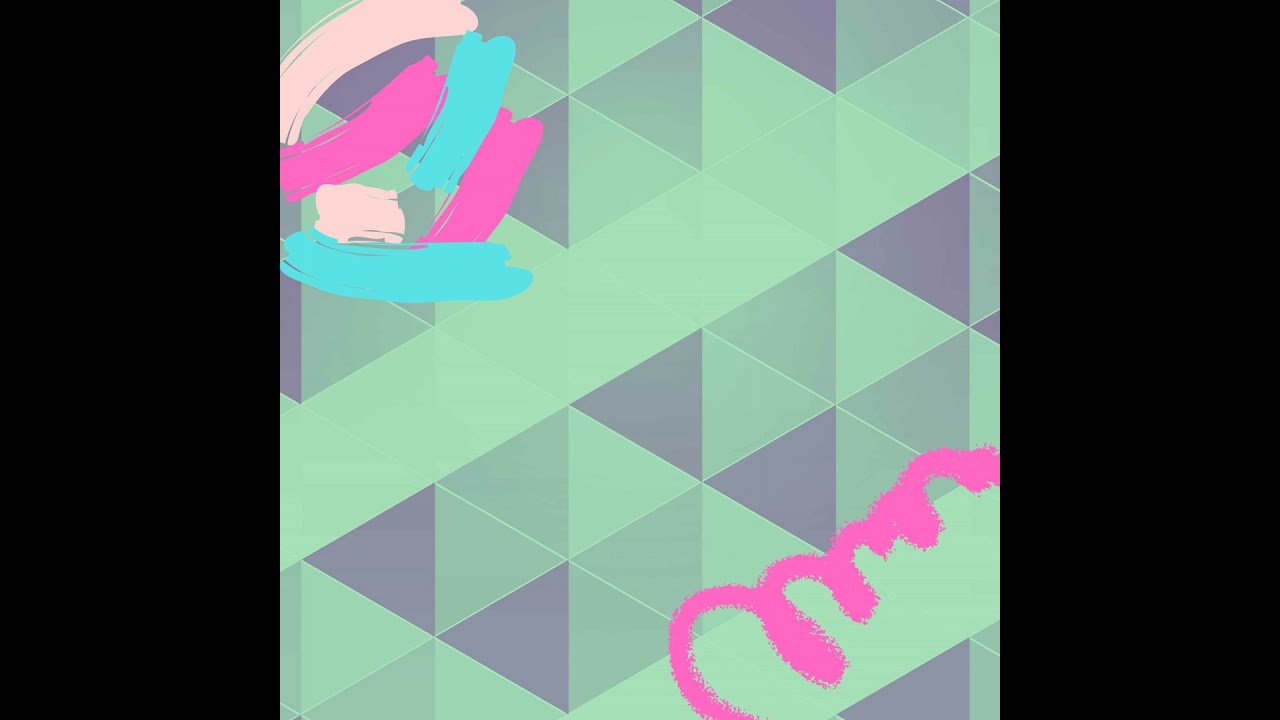The image is a piece of colorful digital art framed within black borders on the left and right, giving it a rectangular shape. Dominated by a mosaic of interlocking, intersecting triangles, the image features a vivid array of colors including mint green, purple, magenta, light blue, light pink, and gray. The triangles are aligned diagonally, creating an optical illusion of cubes and cylinders. In the top left corner, there are paint strokes of light pink, fuchsia, and bright blue, while the bottom right corner showcases a spray-painted magenta squiggle. The overall style merges geometric precision with expressive, freeform brushstrokes.